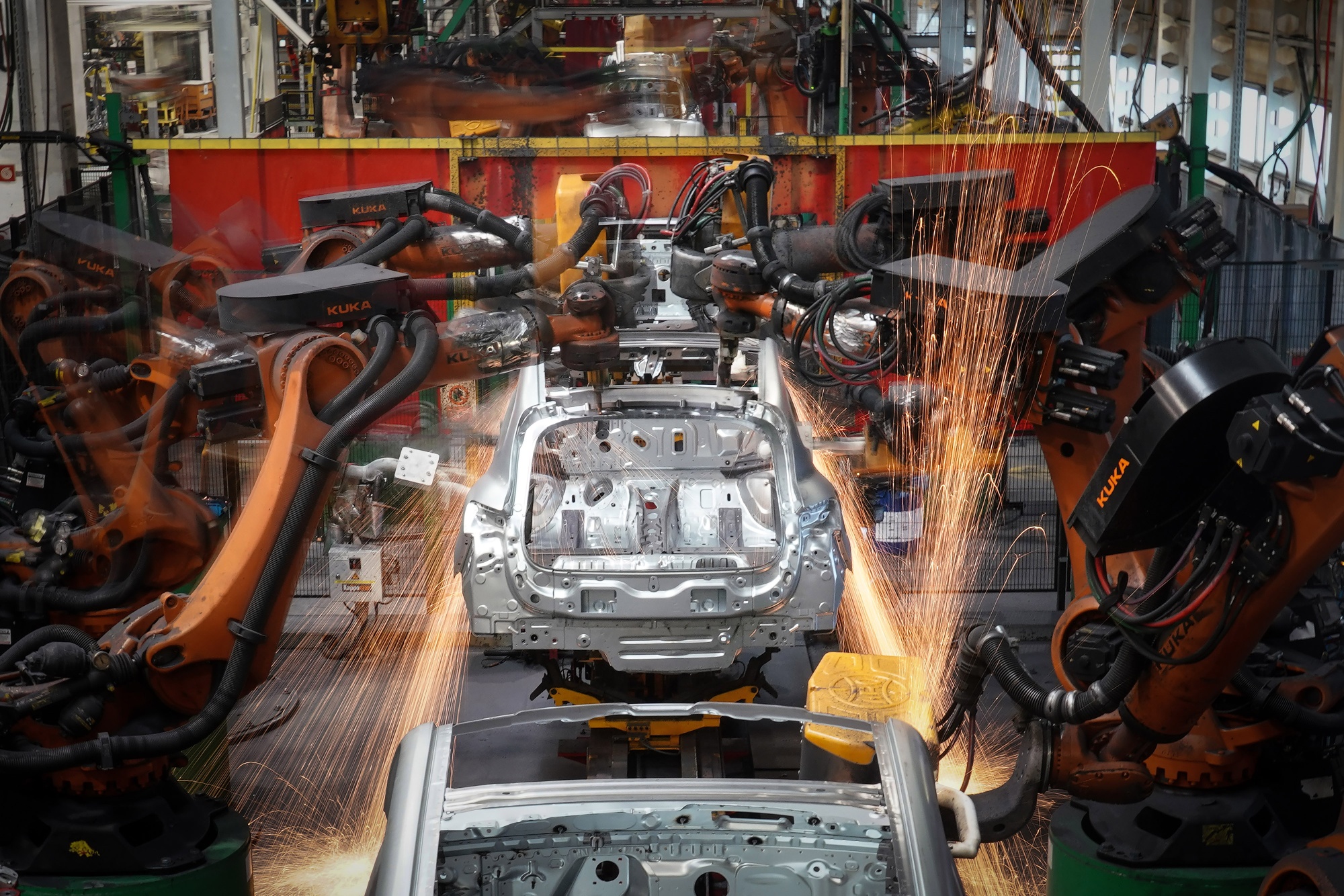The image vividly depicts a bustling car factory assembly line, prominently featuring a series of silver car chassis being meticulously assembled by robotic machinery. On either side of the line, multiple robotic arms, branded with the KUKA logo, are equipped with various attachments and connected by a complex network of black hoses and tubes. These arms are actively engaged in welding operations, sending bright orange-yellow sparks flying both upward and downward, indicating intense fabrication processes on both sides of the frame.

In the center, the unfinished, unpainted metal parts of the cars are positioned, suggesting a dynamic, ongoing assembly procedure. The background reveals a distinctive red wall with a yellow stripe at the top. This wall appears to delineate different sections of the factory, as one can glimpse more machinery and assembly operations continuing behind it.

To the left side of the image, a glass viewing room provides a vantage point over the production activities, enhancing the industrial atmosphere of the scene. The factory setting is further characterized by the visible warehouse space, which is vast and filled with additional machinery equipment, underscoring the scale and efficiency of the automated manufacturing process.